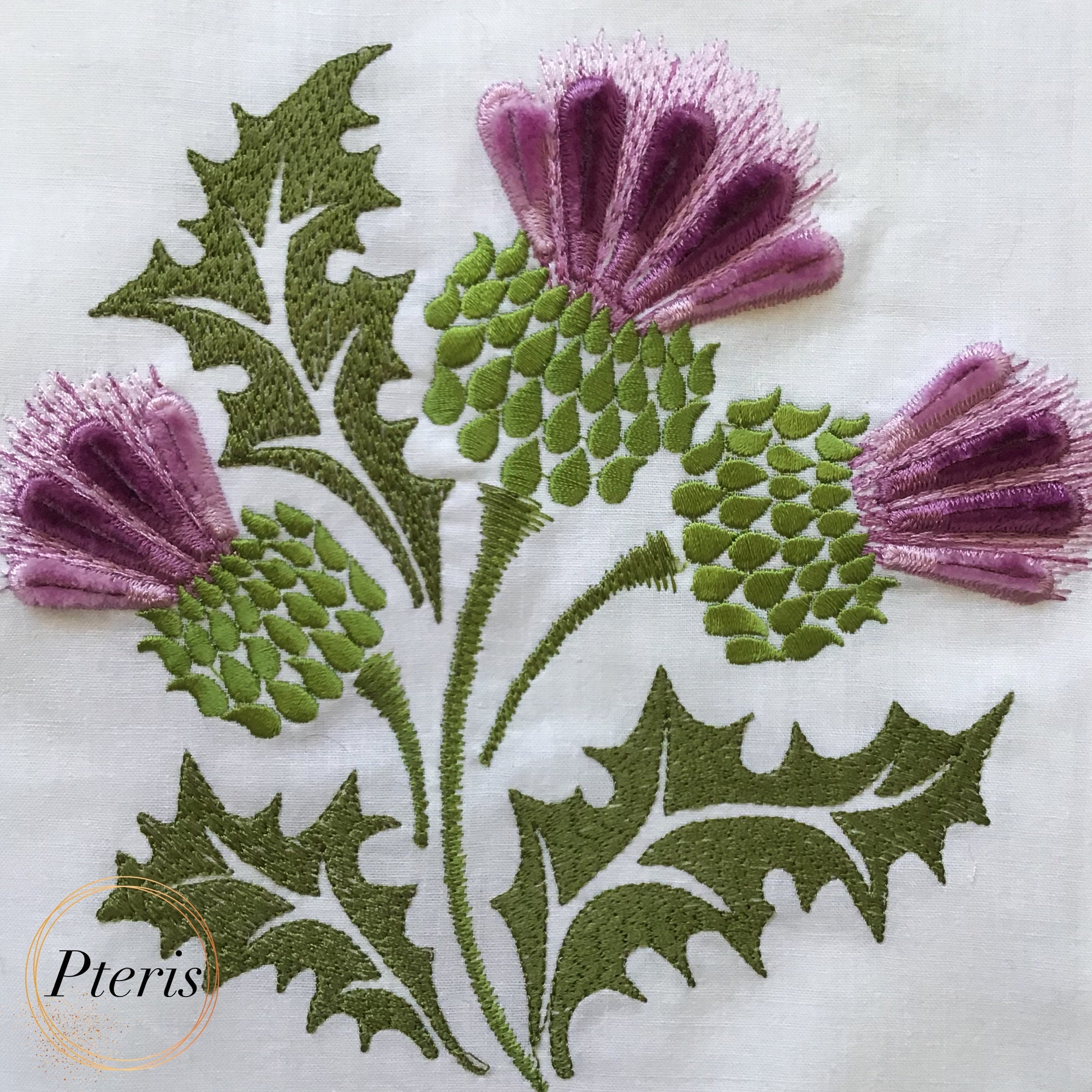This image showcases an elegantly embroidered piece on a white fabric, displaying a meticulous bouquet of flowers. Centralized on the fabric are three curved, green stems that extend upwards, adorned with three large, holly-like leaves and clusters of drop-shaped buds. The embroidery features a rich palette of greens — an olive green with lighter green variations. The main focus is three flowers positioned atop the stems, each boasting intricately elevated and slightly three-dimensional petals in shades of dark and light purple. The sophisticated arrangement of the flowers, with their delicate, feminine petals, adds to the piece's overall aesthetic charm. In the bottom left-hand corner, a gold circle is embroidered with the italicized word “pateris” in black letters, whose meaning remains ambiguous.